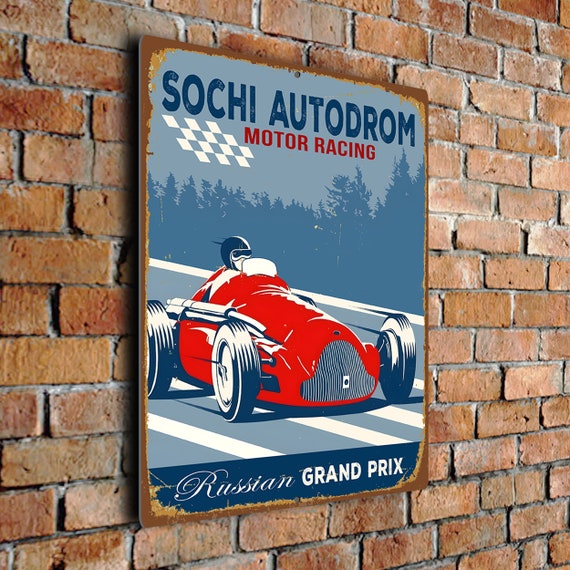The photograph captures a distressed and vintage-style metal sign affixed to a rustic, brown-bricked wall. The sign, weathered and rusted around the edges, prominently features the text "Sochi Autodrome" in large blue letters at the top, with "Motor Racing" in bold red letters beneath it. Central to the sign is an image of an old-fashioned red race car with a notably low and sleek body, exposed wheels, and an open cockpit. The driver, equipped with a helmet and goggles, appears to be racing down a road marked with white lines. Surrounding the car is a forested background rendered in various shades of blue, creating a stark contrast against the car’s vibrant red. Additionally, a blue and white checkered pattern, resembling a racing flag, enhances the poster's racetrack theme. At the bottom, in stylistic white script, it reads "Russian Grand Prix," signifying a race event, with a darker blue background that frames the text. Overall, the image exudes a nostalgic racing atmosphere, emphasizing both the vintage car and the historic racing venue.